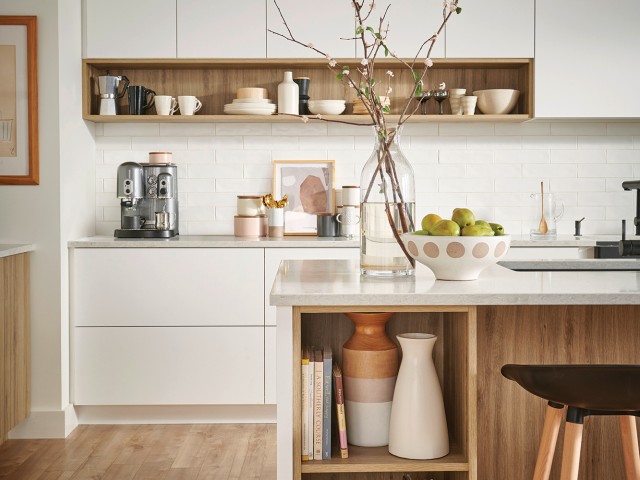This image captures the interior of a modern, mid-century style kitchen predominantly featuring shades of white and light brown wood. The white cabinets have a sleek, handle-less design, and a white marble granite island with built-in cabinetry occupies the center. On the island, a bowl with circular patterns contains greenish pears, and nearby, a jar partially filled with water holds plants with sticks and little branches poking out. A single stool is positioned next to the island. The back counter hosts a variety of items, including a coffee maker, utensils, cups, and a peculiar rock-like painting with a wooden frame. Shelves display an assortment of dishes, such as bowls, wine glasses, plates, and something resembling an espresso maker. To the right, a sink is visible, adding to the kitchen's functional yet aesthetically pleasing design.